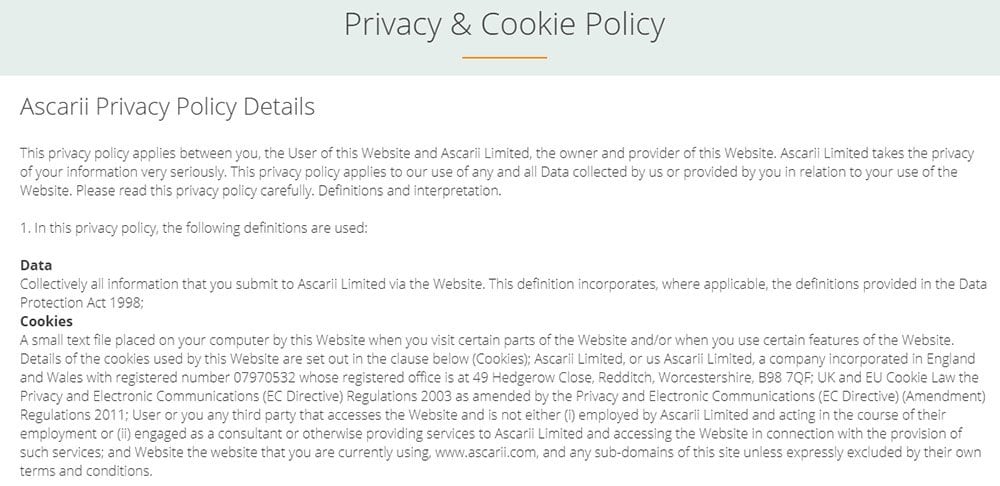The image showcases a detailed view of a SCARI privacy policy document. At the top, the title "Privacy and Copy Policy" is prominently displayed, underlined by a distinctive yellow line for emphasis. The document elaborates on various aspects of the privacy policy, including the types of data collected and the use of cookies, described as small text files that enhance the user experience. Specific sections within the document meticulously outline the data collection process, though only two types of data are explicitly listed.